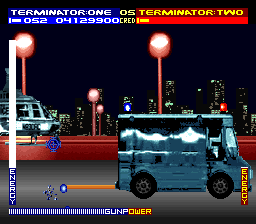In the foreground of this computer game scene, a helicopter is positioned on the left-hand side. The helicopter's front portion, primarily visible, is rendered in shades of white, black, and grey. On the right-hand side, a large rectangular vehicle, resembling an armored security truck typically stationed outside banks, is prominent. This vehicle features reinforced panels and a robust design, colored in grey and black hues. The street beneath the helicopter has a distinctive red coloring, while the road under the armored vehicle is a dark greyish-black.

The background reveals a cityscape with towering skyscrapers, some of which have illuminated windows, adding to the urban ambiance. Additionally, street lights hang above the red-colored street where the helicopter is stationed, casting a red glow downwards, enhancing the scene's atmospheric detail.